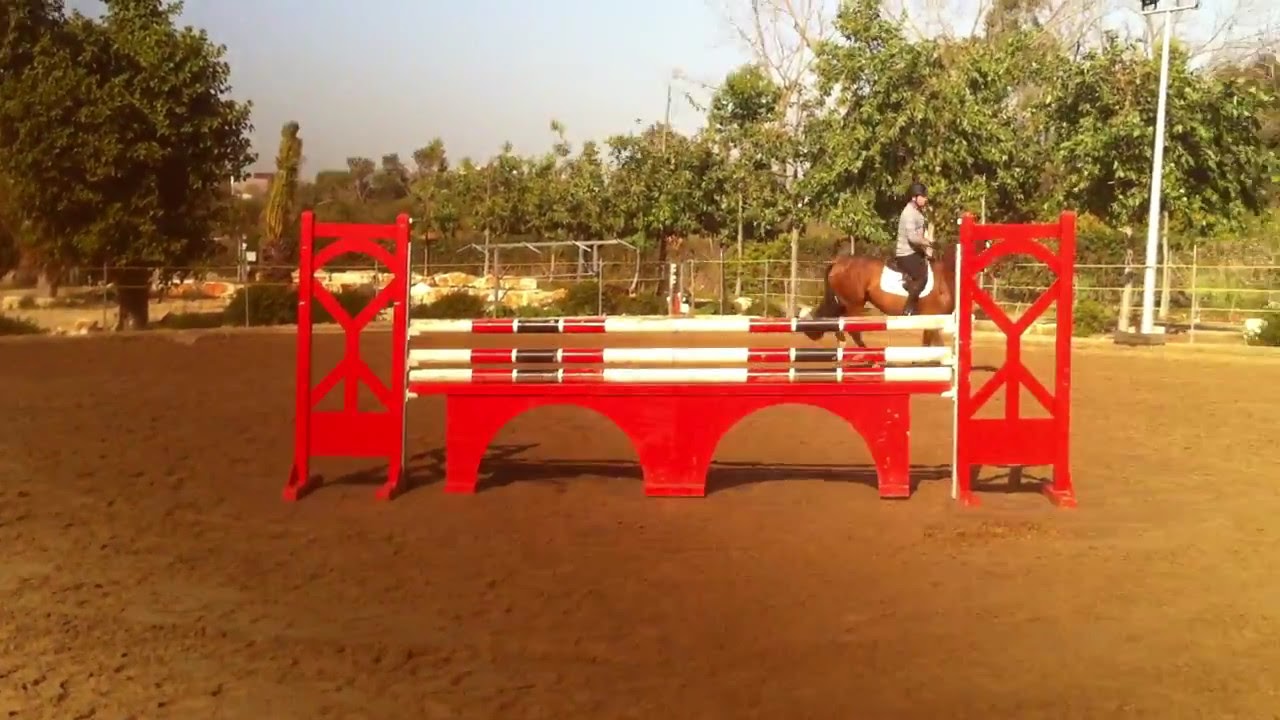This horizontally aligned rectangular photograph captures an outdoor dirt arena framed by a white metal fence. In the background, trees border the fenced area under a mostly cloudy sky, with patches of blue visible, particularly toward the left. Central to the image is a horse jumping obstacle featuring two vertical red posts supporting three horizontal poles painted red, black, and white, arranged in a sequence. A rider, clad in a light-colored long-sleeved shirt, black pants, and a black helmet, sits astride a brown horse partially obscured by the obstacle. The rider's gender is ambiguous, although one account suggests a woman in her 30s. The arena also includes a light fixture on the right side, suggesting nighttime practice capability.